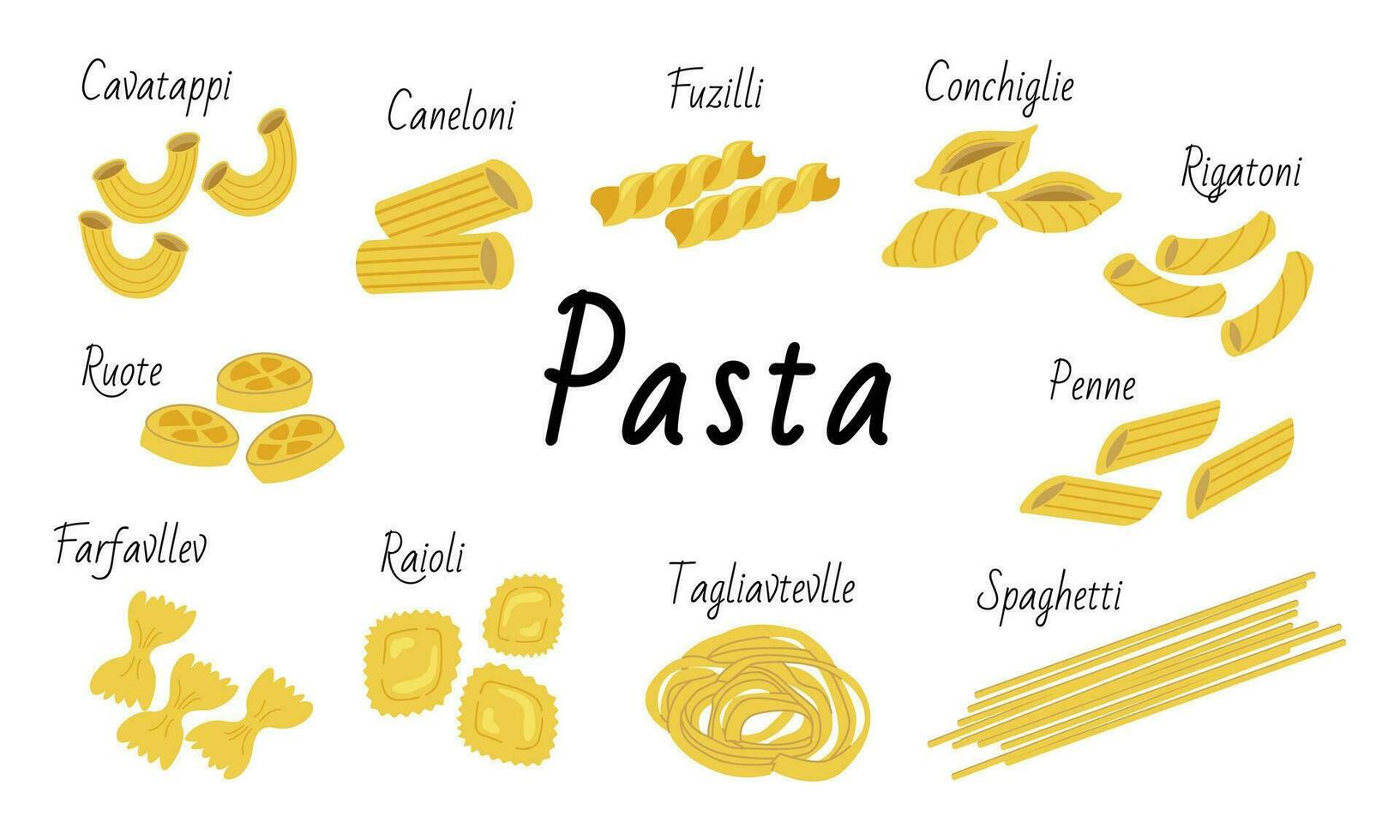This image is a detailed diagram of various pasta shapes against a white background. At the center of the diagram, the word "PASTA" is prominently displayed in bold black letters. Surrounding this central label are images representing different types of pasta, each portrayed in a yellow color to signify the actual pasta shapes. 

Starting from the upper left corner, the pasta labeled "CABOTAPPY" is depicted in black letters. Directly below this, another pasta type labeled "ROUTE" is displayed. Continuing downward, "FARFELY" appears beneath "ROUTE." To the right of "FARFELY," we find the label "RAVIOLI." Moving further right, the word "TAGLIATEL" is positioned next to "RAVIOLI."

In the bottom right corner, "SPAGHETTI" is labeled, and above "SPAGHETTI," the "PENNE" label is placed. Ascending from "PENNE," the diagram shows "RIGATONI" at the top right corner. Moving left from "RIGATONI," "SHELLS or CONGELES" is labeled, with "FUSILLI" situated next to it.

Each type of pasta is depicted in its corresponding shape, accurately labeled by the words above or adjacent to it, collectively creating an illustrative and informative guide to different pasta varieties.